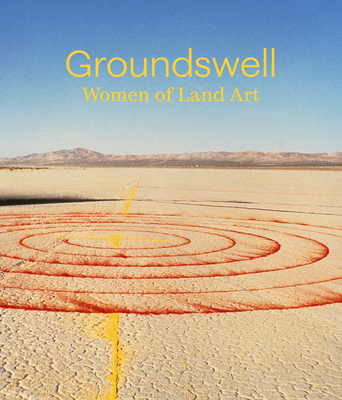The image, evocative of a book cover titled *Groundswell, Women of Land Art* written in yellow text at the top, captures a striking piece of land art set in a stark desert landscape. The expansive, cracked desert soil foreground extends toward a distant mountain range under an unblemished blue sky. Dominating the scene are bright red concentric circles, seemingly formed from sprinkled powder, which spread outward in a captivating spiral, possibly influenced by desert winds. Intersecting these red formations is a prominent yellow line with a perpendicular short line, adding geometric contrast to the organic flow of the circles. A faint black shadow appears in the upper left, hinting at the passage of time or the presence of unseen elements within this barren yet artistically transformed environment.